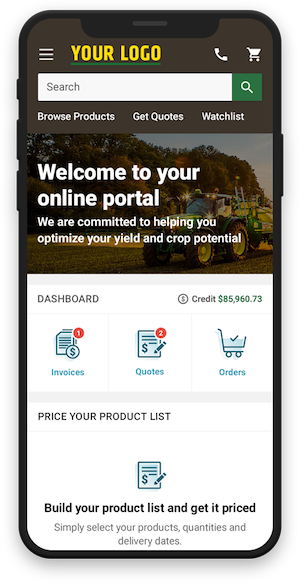The image features a sleek interface designed for an online agricultural portal, set against a black background. At the top, there are three slim white lines accompanied by a yellow "Your Logo," a phone icon, and a shopping cart icon. Below this header, a search box with a green accent and a magnifying glass symbol is present, inviting users to "Browse Products," "Get Quotes," and view their "Watch List."

Dominating the center is an appealing image of a tractor, overlaid with the text, "Welcome to your online portal. We are committed to helping you optimize your yield and crop potential." This welcoming message sits just above a white dashboard box.

Within this dashboard box, key financial details are displayed. On the top-left, a circular icon with a dollar sign denotes available credit, amounting to $85,960.73. Below this, an "Invoices" section marked with a red circle and the number 1, indicating pending tasks, also features a dollar sign icon.

Adjacent to it, the "Quotes" section showcases a red circle with the number 2, and "Orders" is marked by a shopping cart icon with a check mark. The dashboard continues with another white box labeled "Price Your Product List," featuring a list icon, a dollar sign, and a pencil. Instructions read, "Build your product list and get it priced. Simply select your products, quantities, and delivery dates."

This comprehensive portal layout clearly emphasizes user navigation and essential functions, ensuring that all necessary information is readily accessible for optimal agricultural management.